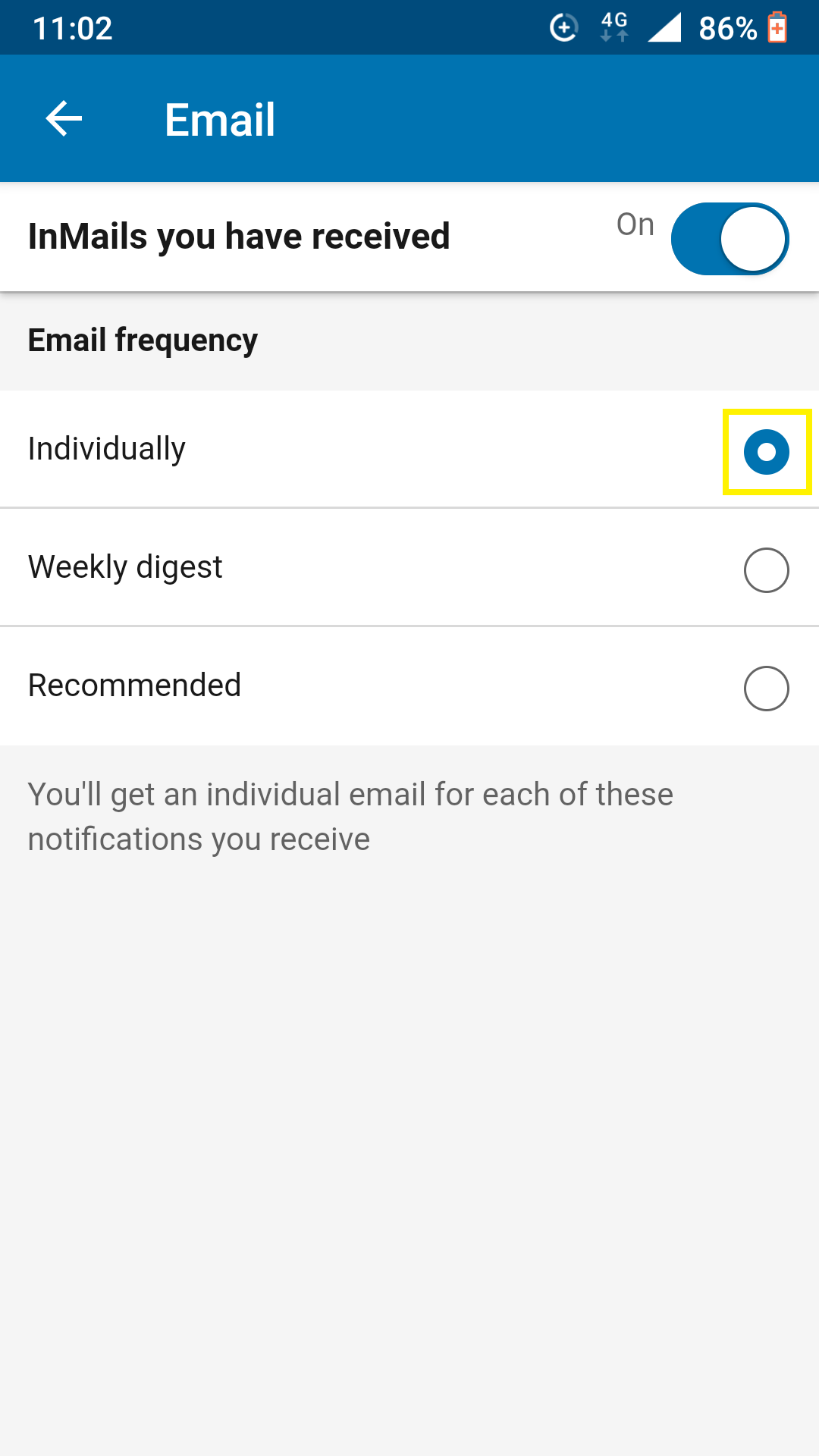Screenshot of the Email Notification Settings Page: This detailed and minimalistic screenshot displays the email notification settings for an application, likely LinkedIn based on the terminology. At the top, a blue header presents the time as 11:02, indicates a 4G network connection, and shows the battery level at 86%. Beneath the header, a back arrow icon and the title "Email" are clearly visible.

The "In Mails You've Received" section appears next, featuring a toggle switch set to "On," signifying that email notifications for received in-mails are enabled. Following this, the "Email Frequency" section offers multiple options for users to select how often they receive email notifications; the choices are "Individually," "Weekly Digest," or "Recommended."

Under the email frequency options, there's a note clarifying that selecting "Individually" will send an email for each notification received. The overall design is crisp and contemporary, adhering to modern design principles with a white background and black text. Selections are indicated in blue via toggle switches and radio buttons, with additional yellow highlights for emphasis. The layout is intuitive, ensuring users can easily understand and modify their notification preferences.